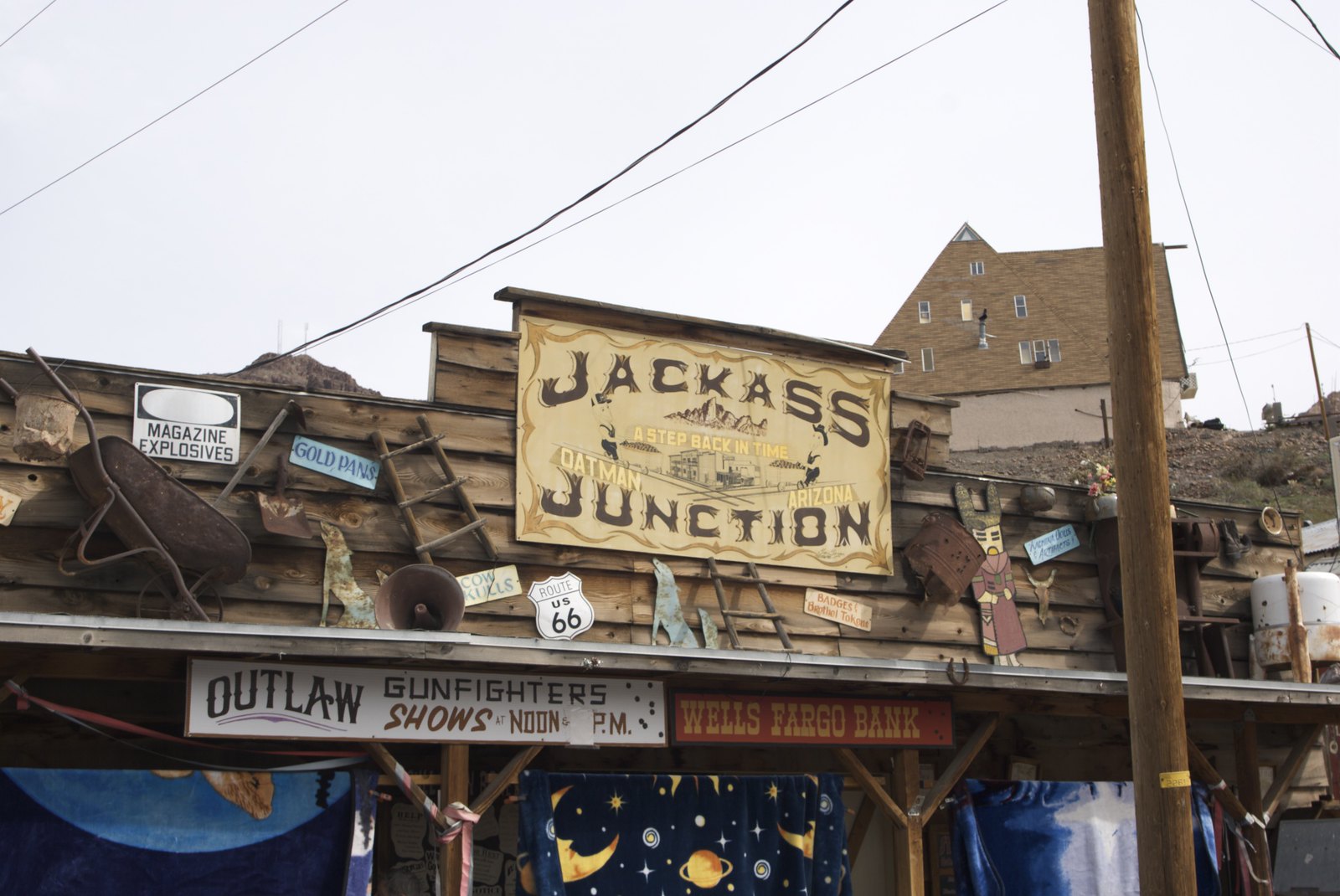The photograph captures a vivid, full-color scene of a storefront in Oatman, Arizona, designed to evoke the nostalgic feel of a Wild West town. The central feature is a prominent wooden sign that reads "Jackass Junction" in dark brown text, accompanied by the phrase "a step back in time, Oatman, Arizona" in yellow letters. Below this, another sign states "Wells Fargo Bank" on a red strip, also displaying "Outlaw Gunfighters Shows" with its showtimes listed at 12 p.m. and 5 p.m. Flanking the sign on both the left and right are additional displays—including a white sign with light brown text reading "Outlaw Gunfighters" and various Wild West-themed elements such as badges, brothel tokens, cow skulls, and gold pounds. There is also a Route 66 sign and an intriguing assortment of props like wheelbarrows, old wood ladders, and a whimsical curtain adorned with stars and planets, evoking a wizard’s hat. Dominating the right side of the image is a very tall wooden telephone or electrical pole, adding to the rustic charm of the entire scene. The photograph showcases the architectural details of the building, including a brown shingled roof with windows, and conjures the imaginative essence of a bygone era.